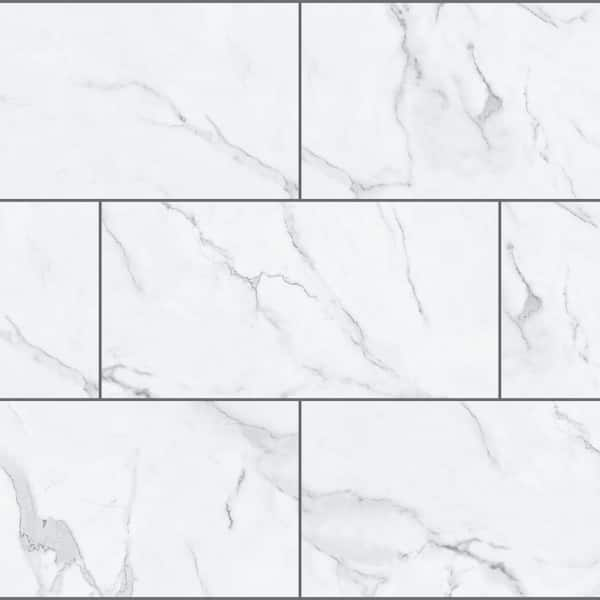This image features a meticulously laid, staggered pattern of white marble tiles, resembling a running bond typically seen in brickwork. Each tile is predominantly white with intricate gray veining, while a few tiles exhibit minimal veining. The grout used is a strikingly stark black, creating a bold contrast against the marble's lighter tones. The layout displayed in the image consists of three rows of tile, each row tightly packed and extending off the frame in every direction. Although the exact application of the tiles is not specified, their dimensions and design make them suitable for use as either a kitchen backsplash or bathroom tiling. The overall craftsmanship suggests skilled installation, with the tiles aligned perfectly and the prominent veining adding an elegant touch to the classic marble aesthetic.